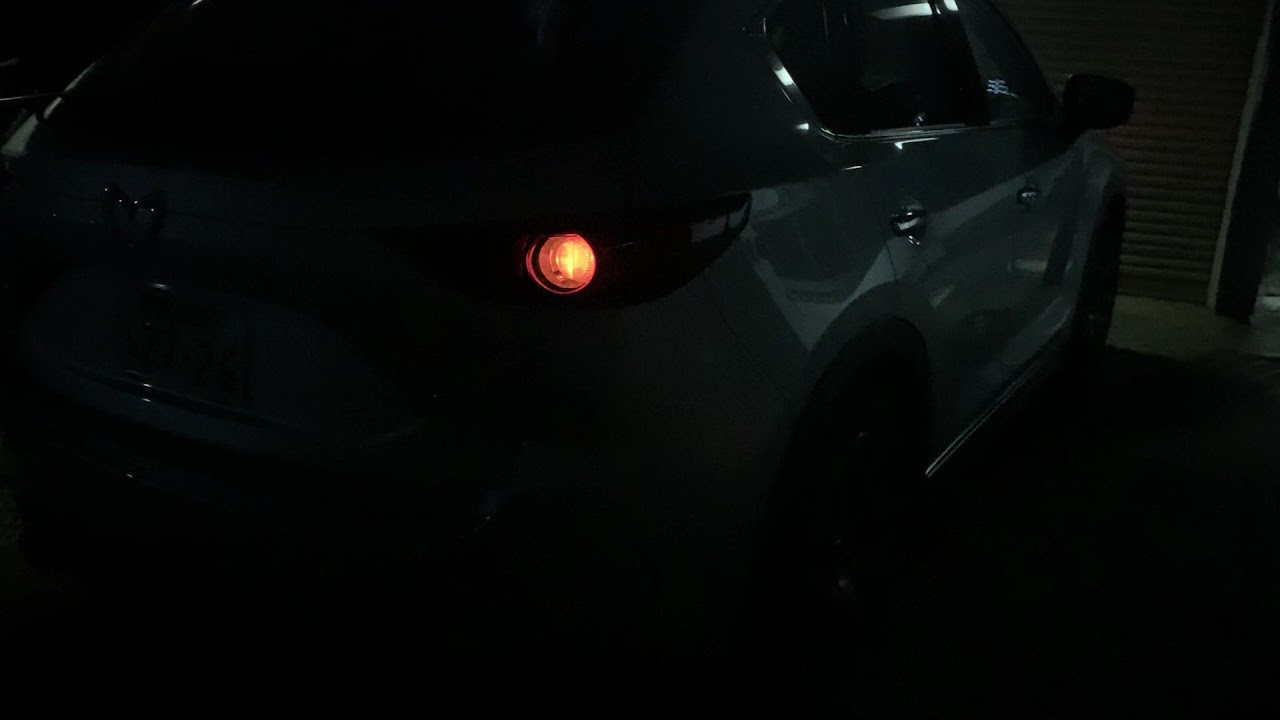In the darkness of a dimly lit garage, a shiny, new light-colored SUV is parked, with the scene defined primarily by the faintly illuminated right taillight at the rear of the vehicle. The SUV's sleek exterior and chrome accents reflect ambient light from overhead garage lights, adding a hint of silver sparkle to its otherwise obscured form. The partially visible scene reveals a closed, metal rolling garage door in front of the vehicle. The taillight, glowing a subdued yellow-orange, draws attention to the passenger side of the SUV, suggesting the brake light is active, and highlights the vehicle's contours that stretch toward the upper left corner of the frame. Despite the pervasive darkness, the image captures the car's modern and pristine appearance.